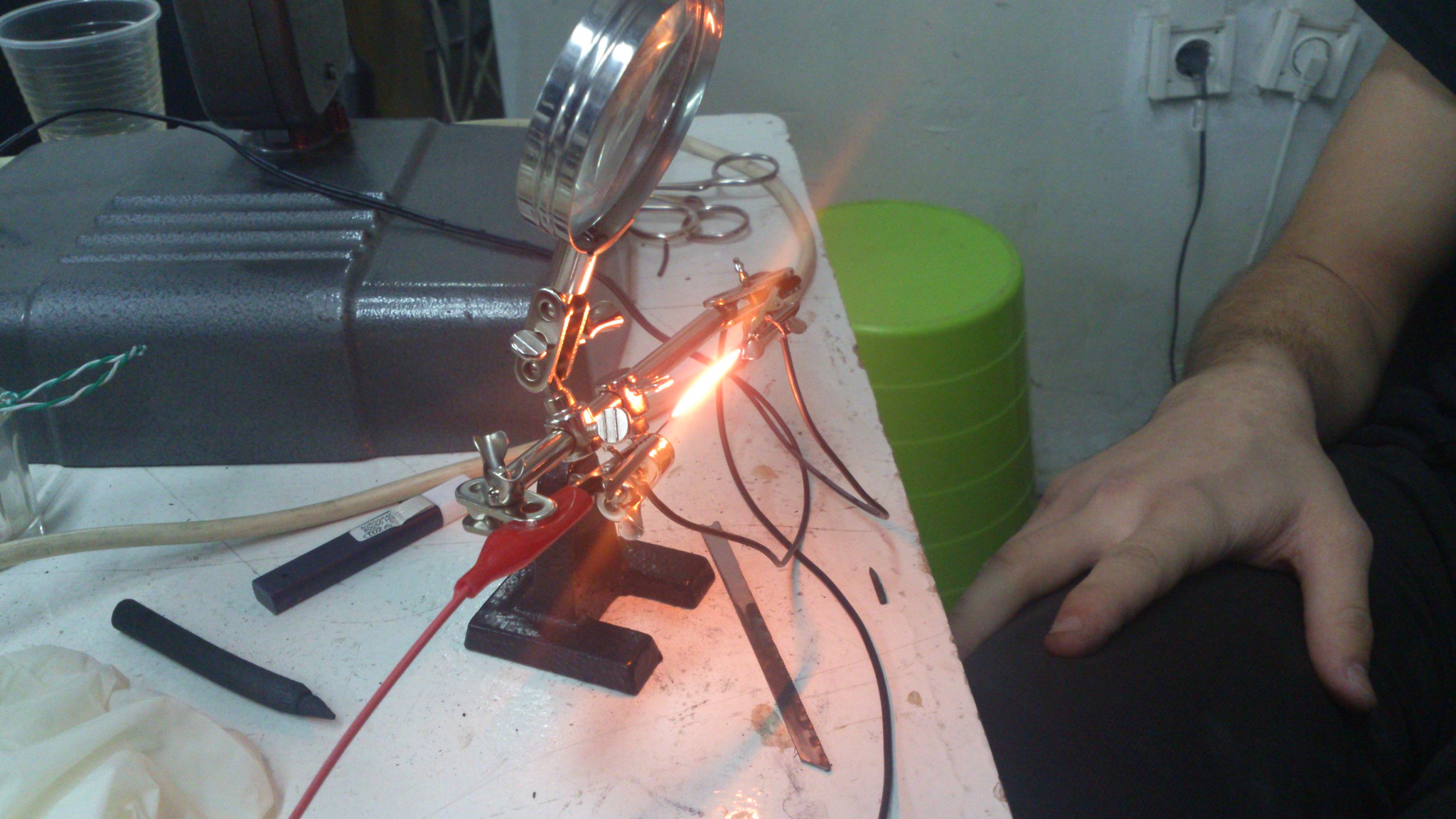In a bustling workshop, a man sits beside a table adorned with various tools and devices. Positioned within easy reach is a large magnifying glass mounted on a black stand. A silver metal bar attached to a red wire and a clear hose takes center stage, with a flame emerging from where the two wires connect. Several smaller black wires branch off each side of the apparatus. The table is strewn with an assortment of items: a black marker or crayon, a used sawzall blade, and a thick, metallic box. At the table's corner sits a clear solo cup, while an upside-down lime green bucket rests in the background. The wall behind features two electrical outlets, one with a white plug and the other with a black plug. The man's arm, resting on his leg, is unpainted and underscores the intense, hands-on nature of his work environment.